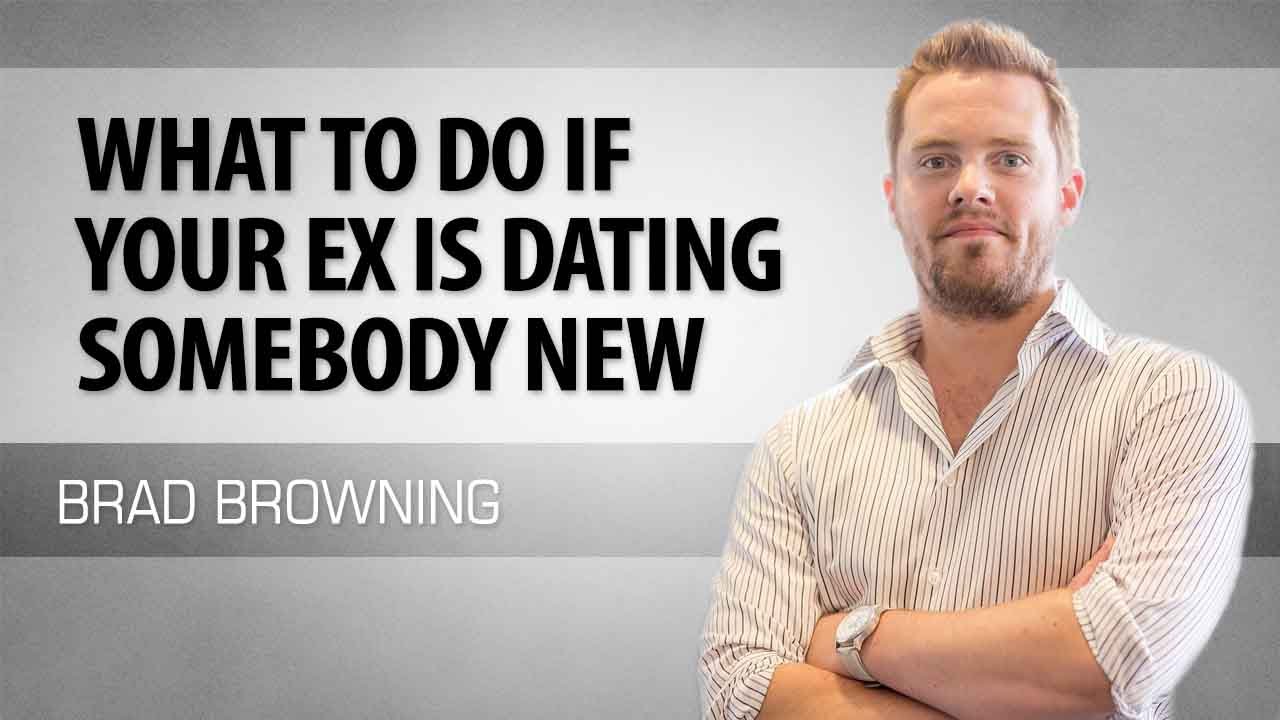The image features a man with short, dark blonde hair that stands up, light brown skin, and thick stubble, giving the appearance of a heavy 5 o'clock shadow rather than a full beard. He has a round forehead and a narrow, elongated face. Wearing a button-down shirt with thin vertical stripes and a silver watch, he stands with his arms crossed over his chest, looking directly into the camera without smiling. The background is predominantly light gray, interspersed with horizontal dark gray bars. Bold, black text on the left side of the image reads, "What to do if your ex is dating somebody new?" Below this text, in white letters against a dark gray bar, is the name "Brad Browning." The composition suggests an educational or entertainment purpose, resembling a YouTube thumbnail or presentation slide. The man is positioned to the right of the image, with all text aligned to the left.